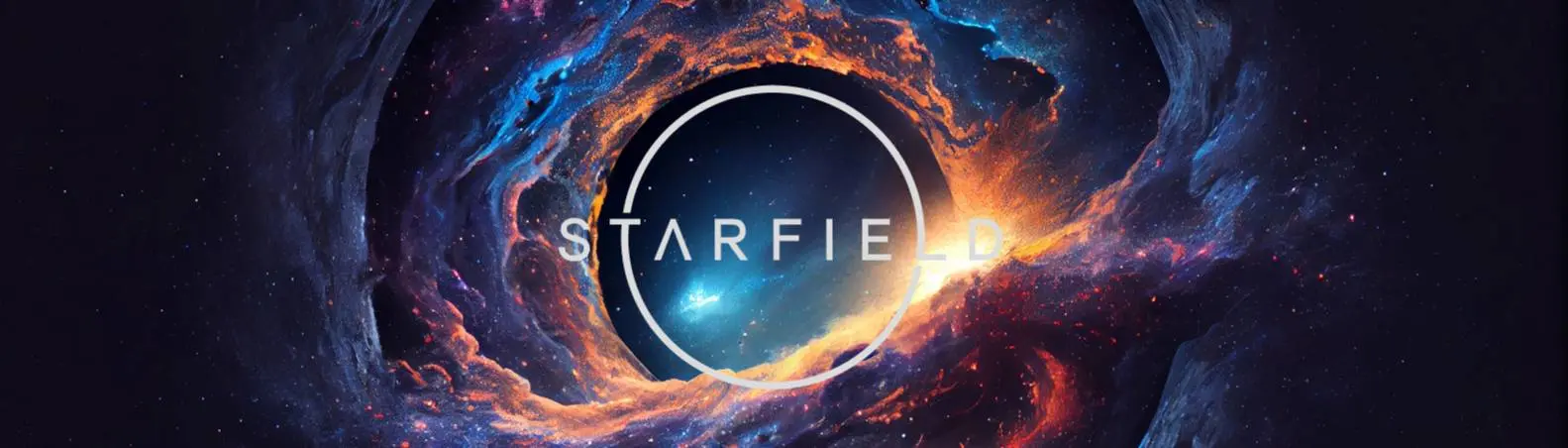This image showcases a stunning depiction of outer space, featuring a central focus on the word "Starfield" written in white. The text is encased within a white circle, with the 'T' and 'L' integrated into the circle's boundary. The arrangement creates a sense of cosmic design, suggesting that it may be from a game or inspired by a space telescope image, such as from the James Webb telescope. Surrounding the text is a vibrant nebula, predominantly composed of red storm-like clouds and interspersed with various colors, including a prominent light blue. The scene is set against a rich star field, with countless stars scattered throughout the background. There's a notable blue light source beneath the letters 'L' and 'D' and a bright section under the 'A' and 'R,' indicative of an intense nebular region. Additionally, a mysterious glowing object can be spotted towards the bottom left of the central circle. This horizontally extensive image captures the awe-inspiring beauty and complexity of a galaxy, presenting a vast tableau of universal wonders.